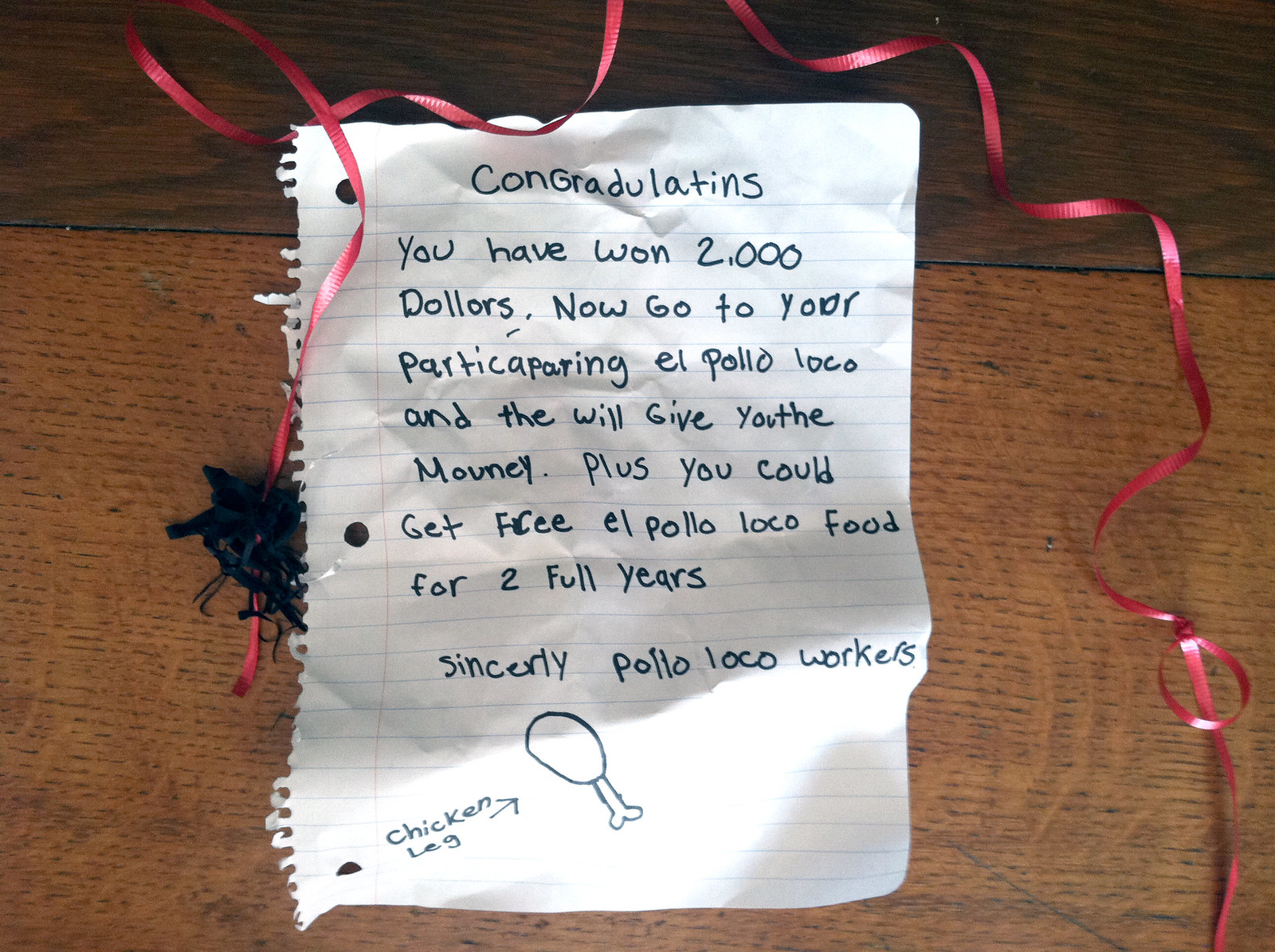The image features a crumpled handwritten note, occupying around 60% of the picture, and set against a brown wooden desktop. The note is written on ragged spiral notebook paper, identifiable by the three-hole punches along one side. Inscribed with black ink, it contains several misspelled words. The note reads, "Congratulations! You have won $2,000. Now go to your participating El Pollo Loco, and they will give you the money. Plus, you could get free El Pollo Loco food for two full years. Sincerely, Pollo Loco workers." Additionally, there is a simple drawing of a chicken leg with the words "chicken leg" and an arrow pointing to it. The note is adorned with a pinkish-red ribbon curled around its edges, suggesting a celebratory theme. However, the overall appearance of the note suggests it might be a prank or a joke due to its informal presentation and spelling errors.